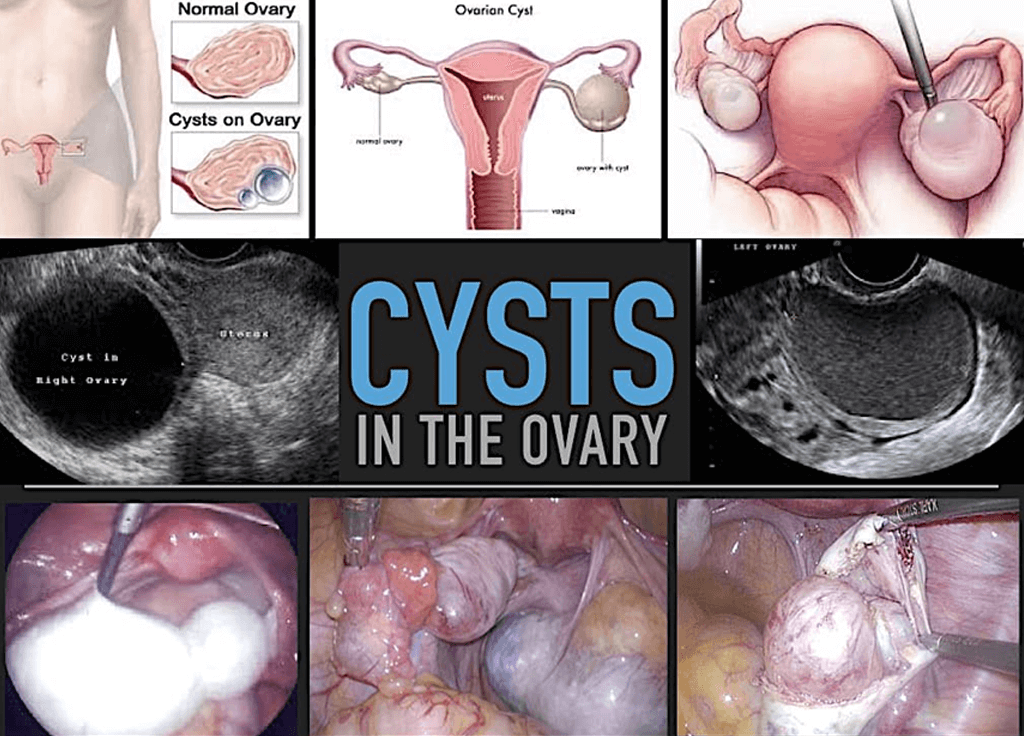The educational image showcases a detailed grid layout illustrating ovarian cysts. At the top, three illustrations depict a normal ovary, an ovary with cysts, and the anatomy of ovarian cysts, each labeled for clarity. The middle section features two black-and-white x-rays, displaying cysts in the right and left ovaries. Between these x-rays, bold blue letters spell out "CYSTS," with "IN THE OVARY" written in white beneath. The bottom row comprises three vivid color photographs from an operating room, capturing real-life images of ovarian cysts being surgically removed. Medical tools are visible, emphasizing the clinical setting and the intricate details of the cysts within the body.